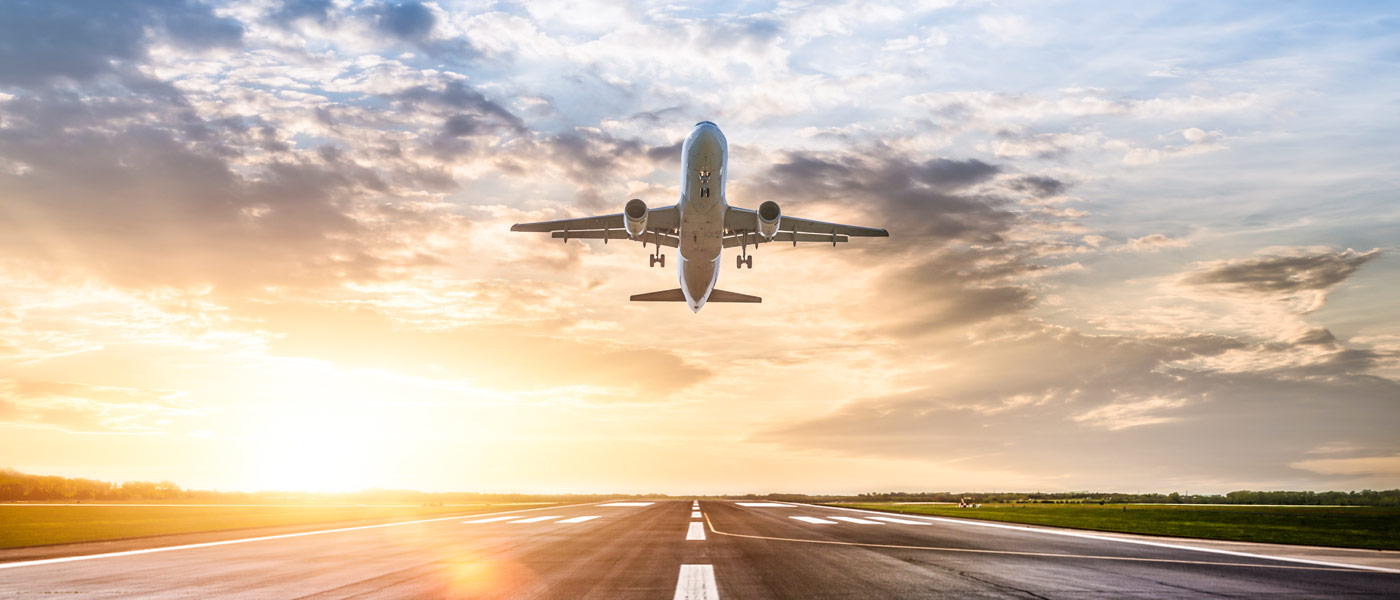The image captures a detailed scene of an airport runway during what appears to be either sunrise or sunset. The grey runway, marked by a continuous white line in the middle, stretches forward and is flanked by bright green grass on both sides. The sky above is a mesmerizing blend of blue, purple, yellow, and orange, with the sun emitting a glowing yellow and white light near the bottom, creating a prominent glare on the runway. Dominating the center of the image is a large, silvery-gray airplane, captured from underneath, either in the initial phase of takeoff or just about to land. The plane has two jet engines, two sets of landing gear extended, and its nose slightly pointed upwards, cutting through a partially cloudy sky. This vibrant and dynamic scene impeccably combines elements of land and sky.